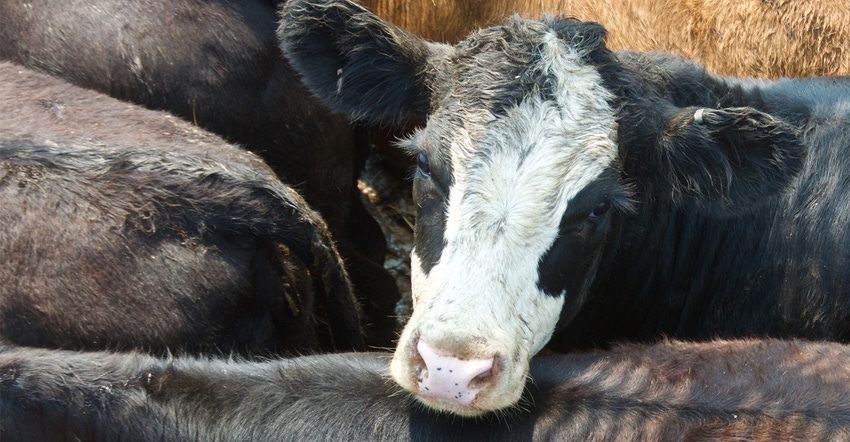This color photograph features the close-up face of a predominantly black cow with some brown accents and a white face, contrasting against his pink nose dotted with dark spots. The cow appears to be looking directly at the photographer with a notably sad expression, its ears drooping to the sides. The cow's head rests on the back of another cow in a tightly packed herd, where only the backs and hindquarters of the surrounding cows are visible. Among these, one cow's back is partially tan and slightly soiled, suggesting a less than pristine environment. The image captures the intricate textures and patterns of the cow's fur, especially the distinctive white patch running down its face and around its nose. In the background, some hay is faintly visible, signifying their rural setting. Despite being surrounded by other cows, the primary focus remains on the face of this single cow, whose sad eyes convey a sense of awareness and melancholy.